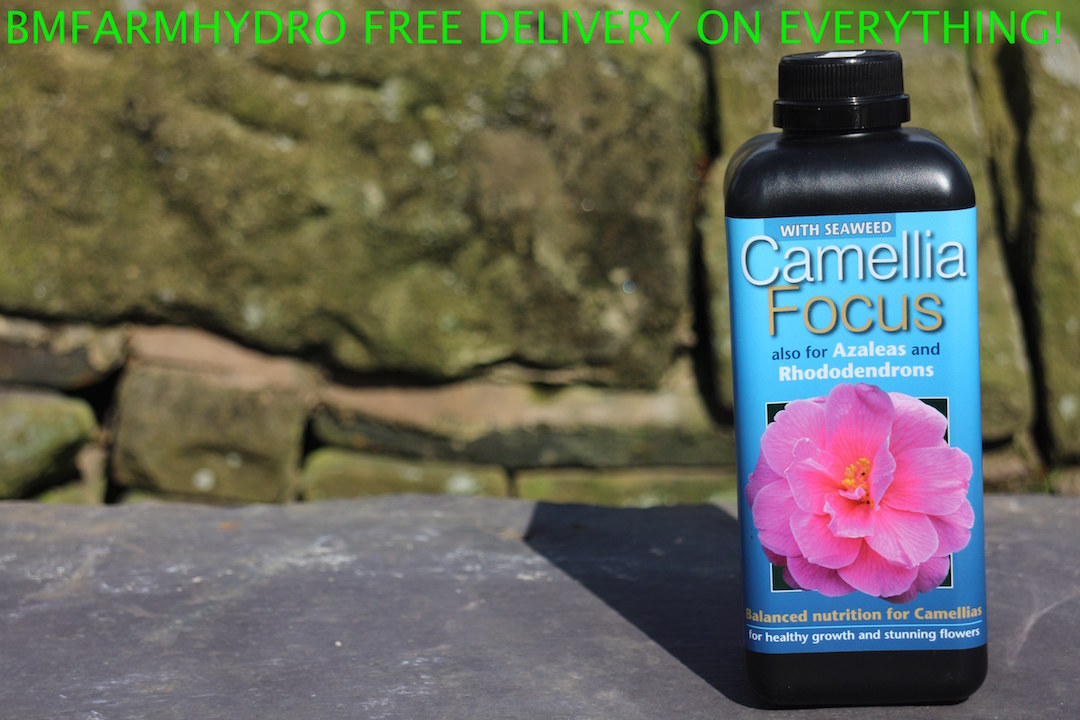This is a detailed outdoor photograph of a black bottle with a label that advertises plant food specifically for camellias, azaleas, and rhododendrons. The label, which shifts from a light turquoise blue at the top to a darker shade of blue towards the bottom, prominently features a vibrant pink flower with delicate petals and visible yellow stamens in the center. Above the image of the flower, the label reads "Whip Seaweed Camellia Focus," emphasizing its use for azaleas and rhododendrons as well. Beneath the flower, the caption in yellow text states "Balanced Nutrition for Camellias," followed by a blue line, under which in white text it promises "For Healthy Growth and Stunning Flowers." The bottle is situated on a gray stone ledge, with its shadow clearly visible, emphasizing the sunny outdoor setting. The backdrop includes a gray stone wall, adding a rustic touch. At the top of the image, bold lime green text declares "BM Farm Hydro Free Delivery on Everything!"